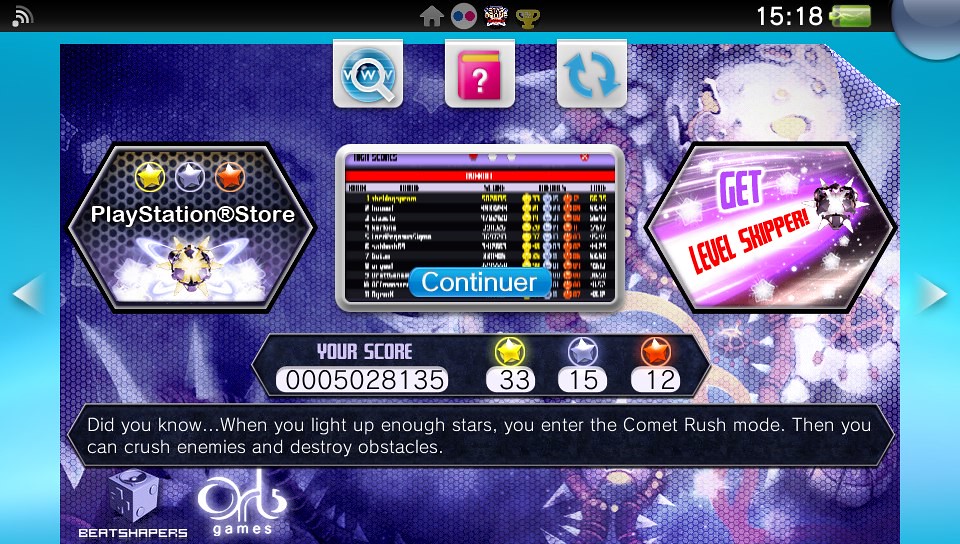The image is a vibrant and colorful screenshot, likely from an old video game system such as the Sony PlayStation Vita. The screen is predominantly light blue with a gradient effect, featuring various modern and colorful icons—a pink book with yellow pages and a question mark for help, a refresh button, a search button, and more. 

At the top, there's a thin black strip displaying the Wi-Fi signal on the left, the time (1518), and a green battery icon on the right, indicating charging. Dominating the center is a large window with a slightly folded upper right corner, displaying several lines of text and scores. The middle section includes a detailed scoreboard showing a score of 5,028,135, with gold stars totaling 35, silver stars 15, and bronze stars 12.

On the left side of this window, the PlayStation Store logo is prominently displayed with three stars above it. The middle section also contains a blue 'Continue' button, while on the right side, there's a button labeled 'Get Level Shipper.' At the bottom, a message reads, "Did you know when you light up enough stars you enter Comet Rush mode? Then you can crush enemies and destroy obstacles." The overall design is dynamic with numerous object shapes and vibrant yellow highlights.